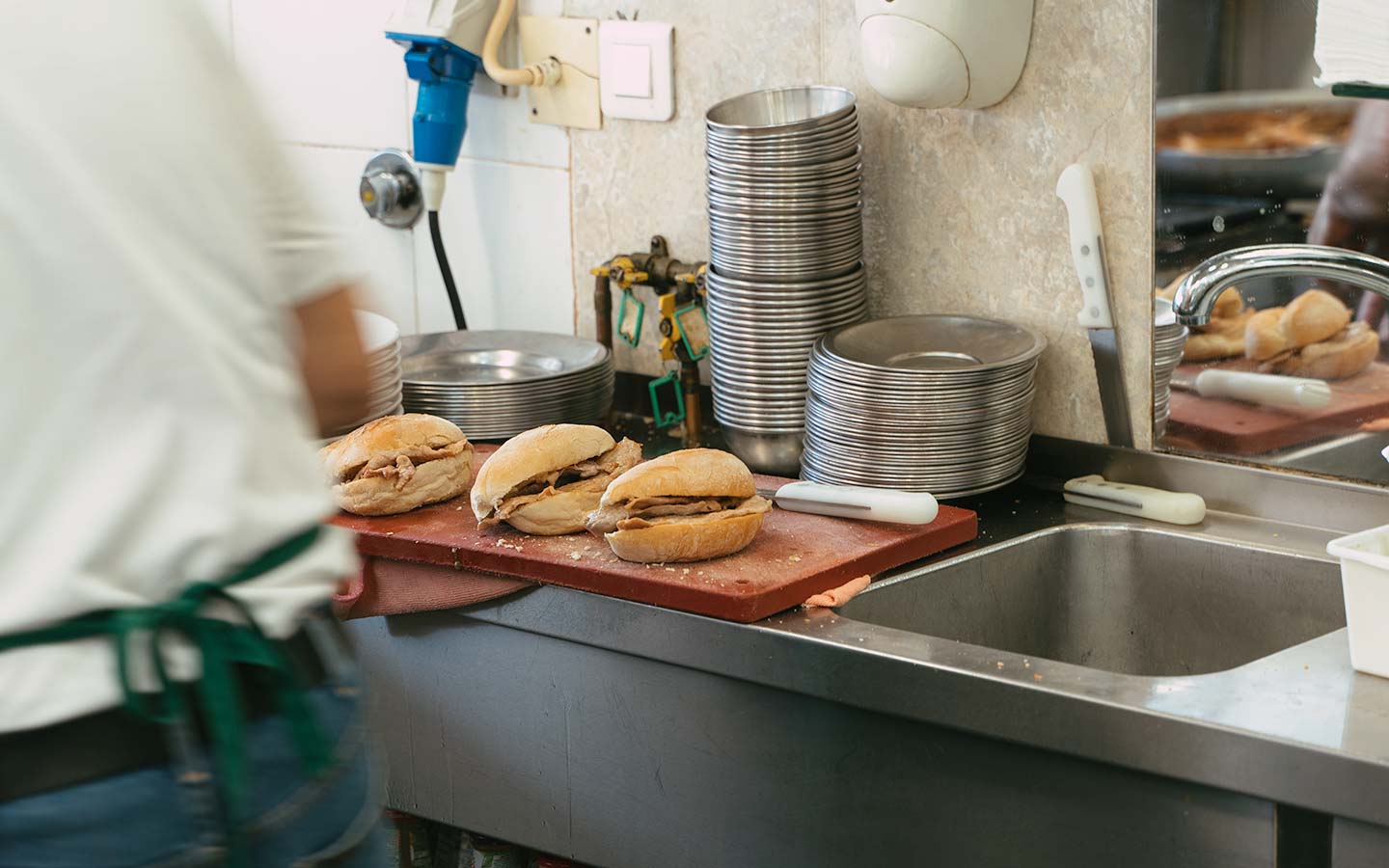In this horizontal photograph of a kitchen, a man is seen from the back, dressed in a white short-sleeve t-shirt, blue jeans with a black leather belt, and a green apron tied around his waist. The scene captures him in the midst of sandwich preparation. To his right is a square stainless steel sink and a gray silver counter. On the counter, stacks of metal silver round plates and bowls are visible, with two stacks of plates flanking a stack of bowls. In front of these is a large maroon plastic cutting board that holds three sandwiches on white rolls, each filled with meat. A knife with a white handle lies on the cutting board. Above the sink, a silver faucet and a mirror reflecting parts of the scene are visible. The kitchen has a beige wall and a mixture of blue, white, and gray elements. The entire image highlights the organized, yet busy atmosphere of sandwich-making in a well-used kitchen.